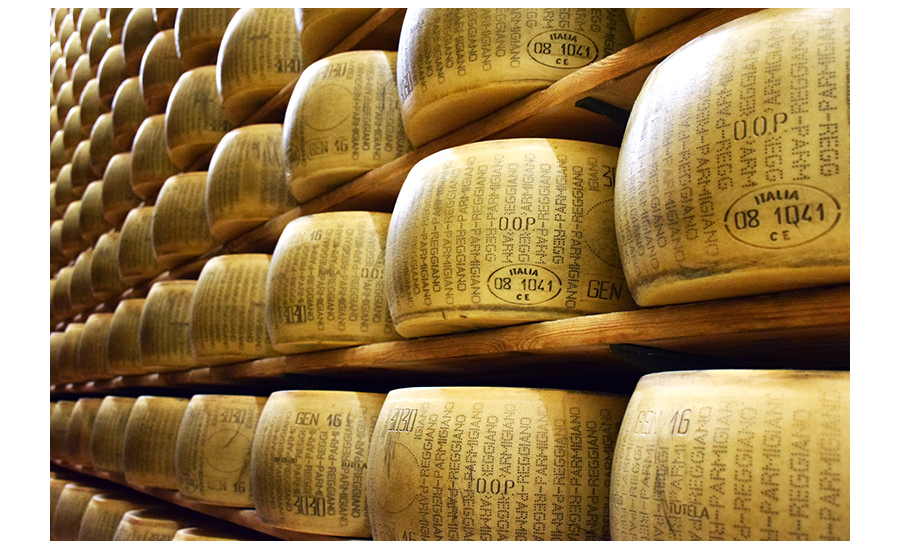This image captures an extensive storage area in Italy, where hundreds of Parmigiano-Reggiano cheese wheels are methodically aged. The cheese wheels, which resemble short, barrel-shaped containers, are meticulously stacked on approximately ten rows of wooden shelves. Each wheel is embossed with a pixelated dot font that reads "Parmigiano-Reggiano," and features an oval label at the bottom marked "Italia" along with a series of numbers, such as "081041CE," as well as additional codes like "Gen 16." These numbers likely indicate production or aging dates, although their exact meanings are unclear. The arrangement of shelves and cheese wheels extends to the left of the image, suggesting a vast and orderly storage system crucial for the aging process of this iconic Italian cheese.